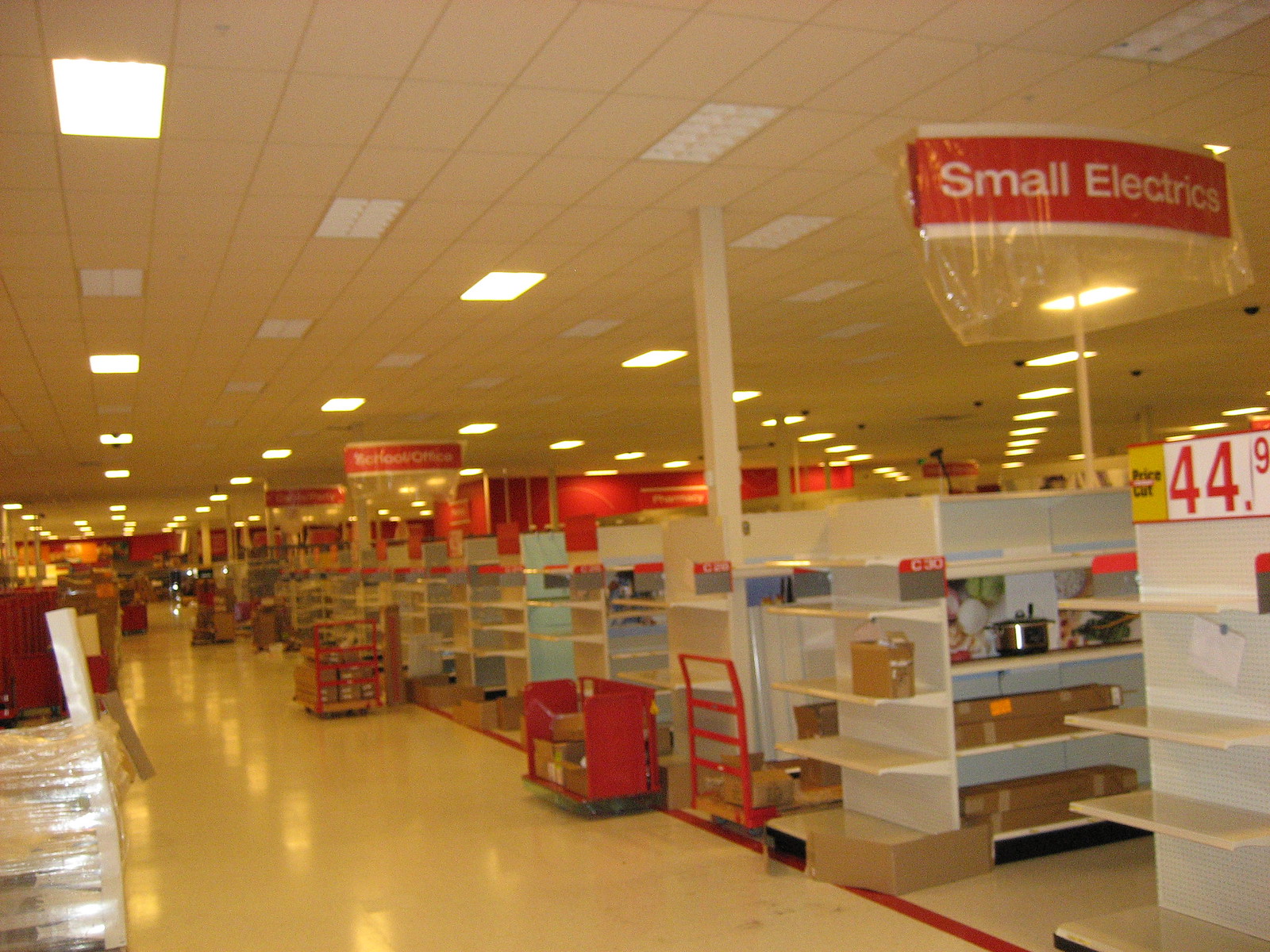The image is a wide-angle, first-person POV color photograph capturing the interior of what appears to be a vintage-looking Target store. The overall scene has a nostalgic feel due to the yellow-tinted lighting that bathes the empty store, adding to the aged appearance. The composition reveals a polished white floor and a tiled ceiling designed in a rectangular grid, interspersed with small square lights.

To the right side of the image, a tall red banner reads "Small Electrics" in white curved text, hanging above one of the mostly empty shelves. A few other red signs, including one indicating a price cut at $44.99 and another mentioning "Office" and "Pharmacy" in the distance, contribute to the sense of a diverse, general retail space.

Numerous stocking carts and dollies are stationed throughout the scene, along with shrink-wrapped pallets visible in the bottom left corner, suggesting the store is either in the process of being set up or restocked. The walkways and aisles are devoid of any people, enhancing the serene and somewhat abandoned atmosphere of the store.